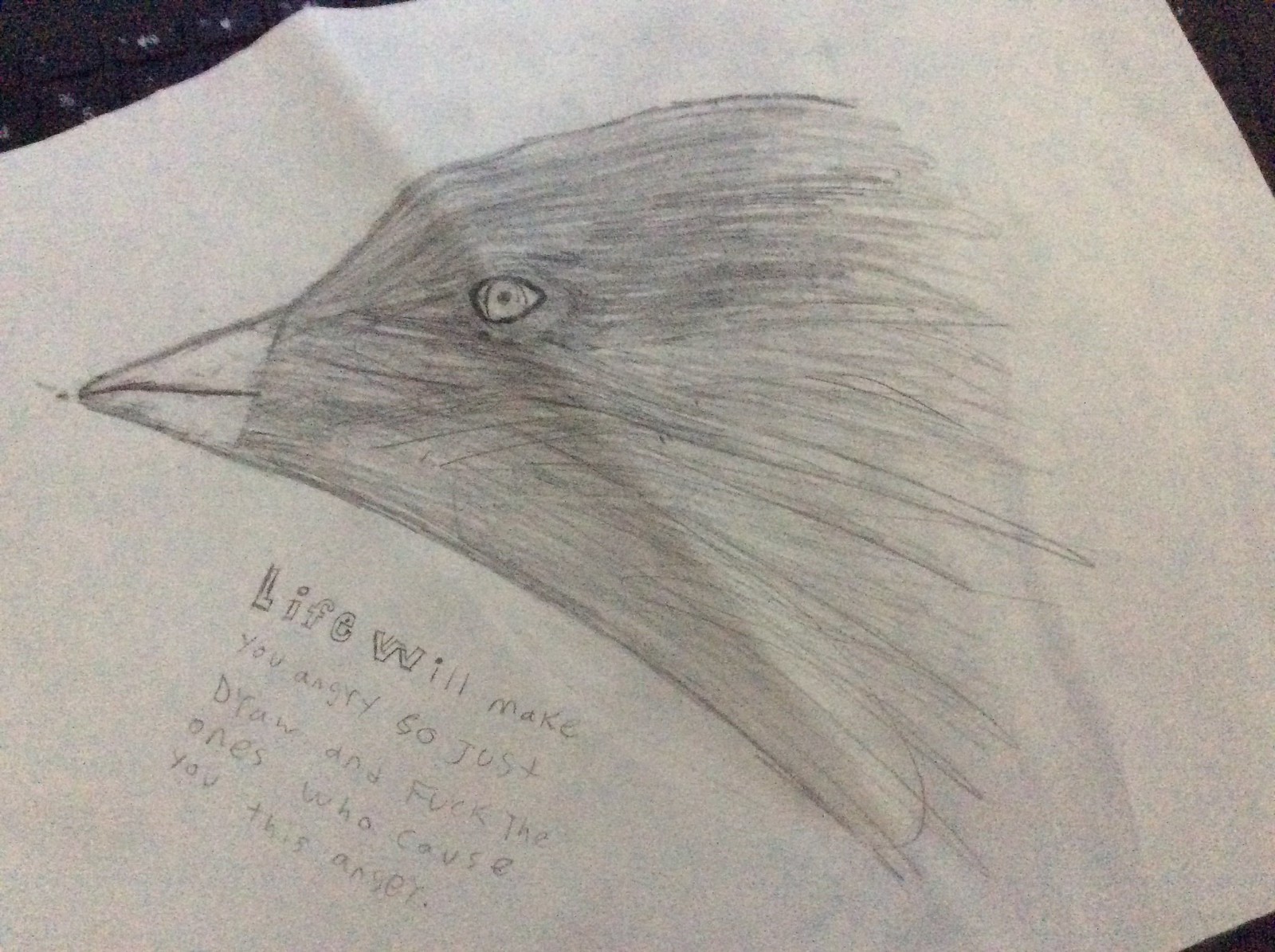The image features a detailed sketch of a crow, predominantly shaded in black pencil, positioned slightly to the left. The crow’s head is the focal point, consuming much of the center of the white, slightly beige paper, due to subpar lighting that affects the color quality. The bird is depicted with a clearly defined beak, an eye looking towards the viewer, and partially extended body feathers. Below the sketch, a bold motivational message, "Life will make you angry, so just draw and fuck the ones who cause you this anger," is handwritten. The paper, slightly tilted, almost fills the frame, lying on a dark surface where parts of a keyboard—including symbols like the percent sign, number five, and a volume button—are visible in the background.